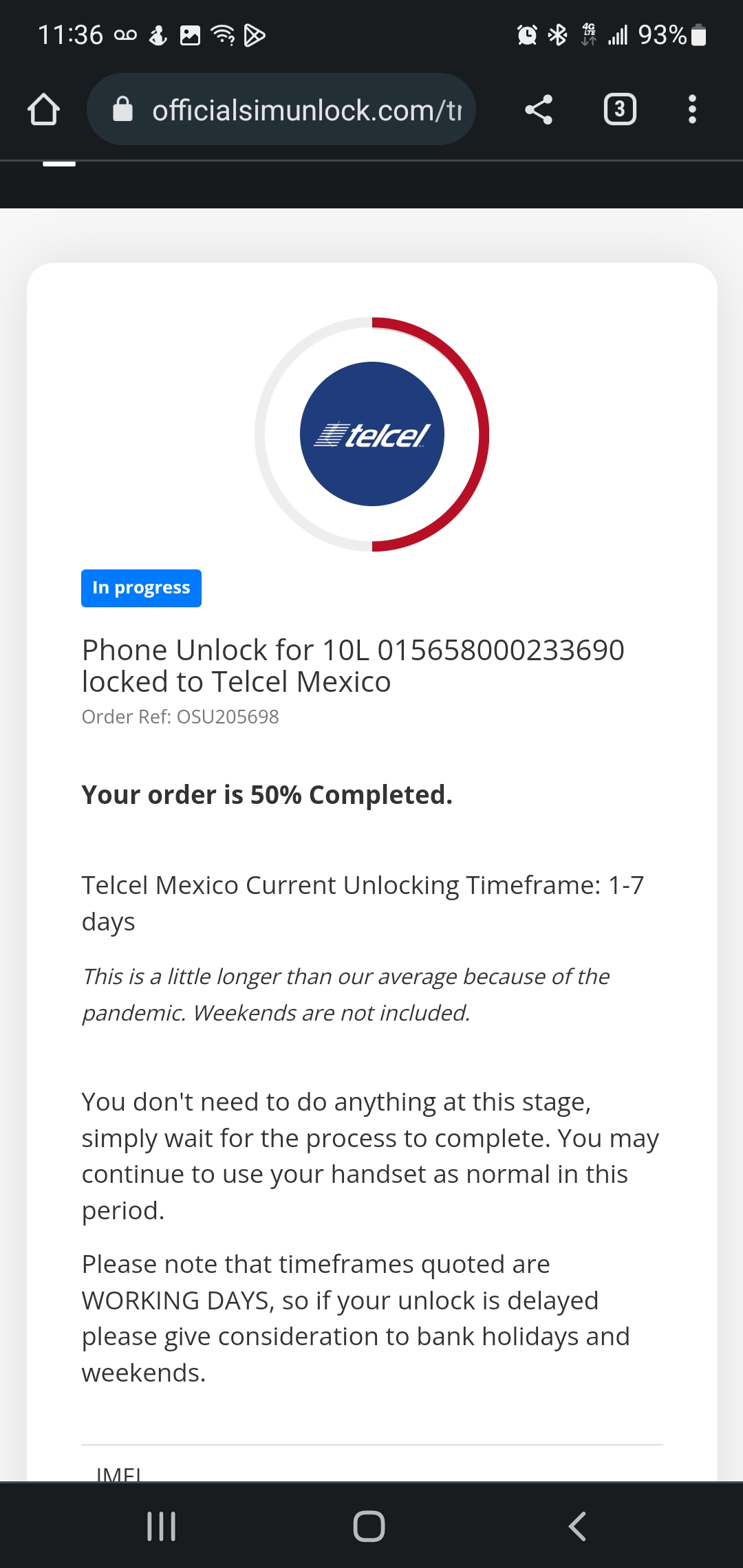Screenshot of a smartphone screen captured at 11:36 AM with various status icons including a 93% battery indicator, four signal bars, and a secure website symbol. The home icon is situated to the left of a URL bar displaying "official.imunlock.com" accompanied by a lock icon indicating a secure connection. The main content section features a light gray border surrounding a white background. Prominently displayed is a dark blue circle labeled "Telcel" and a blue box underneath stating "In Progress". Below that, detailed information reads: "Phone unlocked for 10L01565800233690, locked to Telcel Mexico. Order reference number OSU205698. Your order is 50% completed. Telcel Mexico current unlocking time frame: 1-7 days. This duration is longer than average due to the pandemic; weekends are not included. You do not need to do anything at this stage, simply wait for the process to complete. You may continue to use your handset as normal during this period."